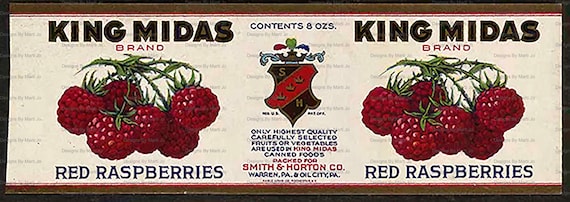The image is a vintage-style advertisement for "King Midas" brand red raspberries, featuring a repeated design on both the left and right sides. Each side displays an illustration of several vibrant red raspberries with small surface details, connected by green stems and topped with tiny green leaves. Above the raspberries, bold black text with a dark gray shadow reads "King Midas," followed by the word "brand" in smaller red text. Below the raspberries, the text "red raspberries" is prominently displayed. An eight-ounce content label is mentioned in blue text. At the center of the label is a crest with a pointed shield, featuring an 'S' and an 'H' in black segments flanking a red stripe adorned with three small golden crowns. Additional blue text states, "only honest quality carefully selected fruits or vegetables are used in King Midas canned foods," and notes the producer as Smith and Hamilton Company, Warren Pennsylvania, Oil City Pennsylvania. The background is predominantly white with a gray border and a smaller red outline at the top and bottom.